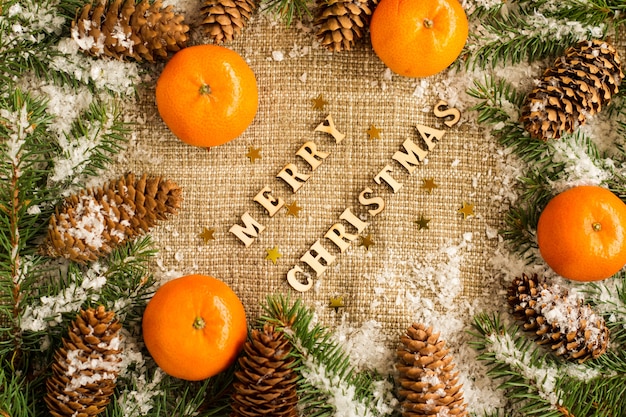The image is a vertically oriented, horizontal rectangle photograph featuring a festive Merry Christmas theme. The words "Merry Christmas" are spelled out in small brown letters at an angle across a burlap bag backdrop. The natural burlap fabric is adorned with pinecones, fir leaves, and a dusting of white sprinkles mimicking snow. Arranged around the photograph are four tangerines positioned at the right, left, top, and bottom of the image. Additionally, there are nine to ten pinecones and eleven golden stars scattered throughout, adding to the festive feel. The overall composition of natural elements and holiday decorations creates a warm, seasonal atmosphere.